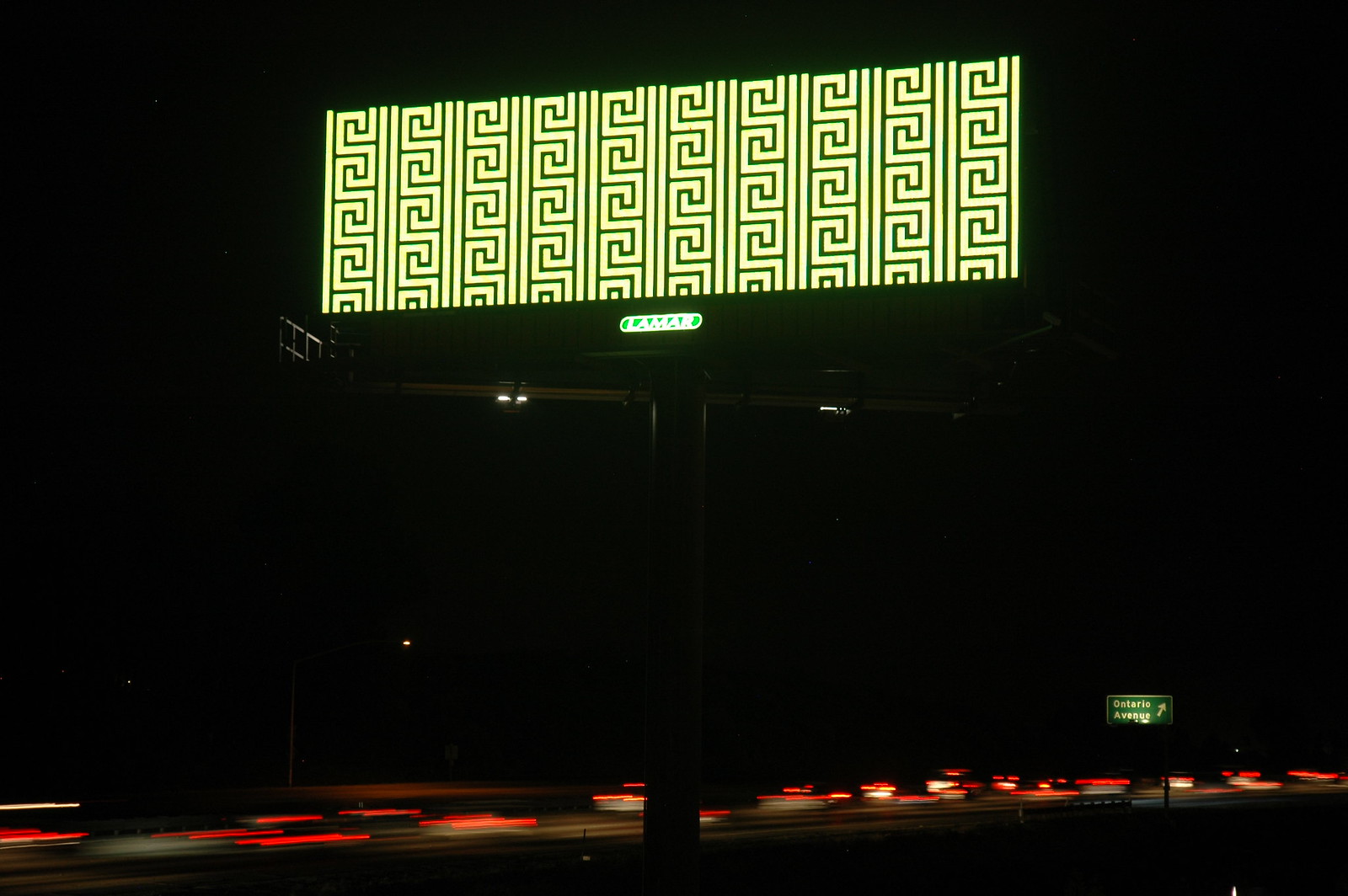The image depicts a dark nighttime scene on a busy road or highway. The majority of the scene is shrouded in darkness, with car red taillights forming a blurry line across the bottom, suggesting vehicles speeding by. In the middle and top section of the image, there is a lit electronic billboard. This billboard features a repeating green geometric pattern on a yellow background and prominently displays the word "LAMAR" in white letters on a long, elongated green oval. Towards the right-hand side of the road, there is a green road sign with white lettering reading "Ontario Avenue" and an arrow pointing to the right. The rest of the image is predominantly dark, with only occasional light spots or reflections.